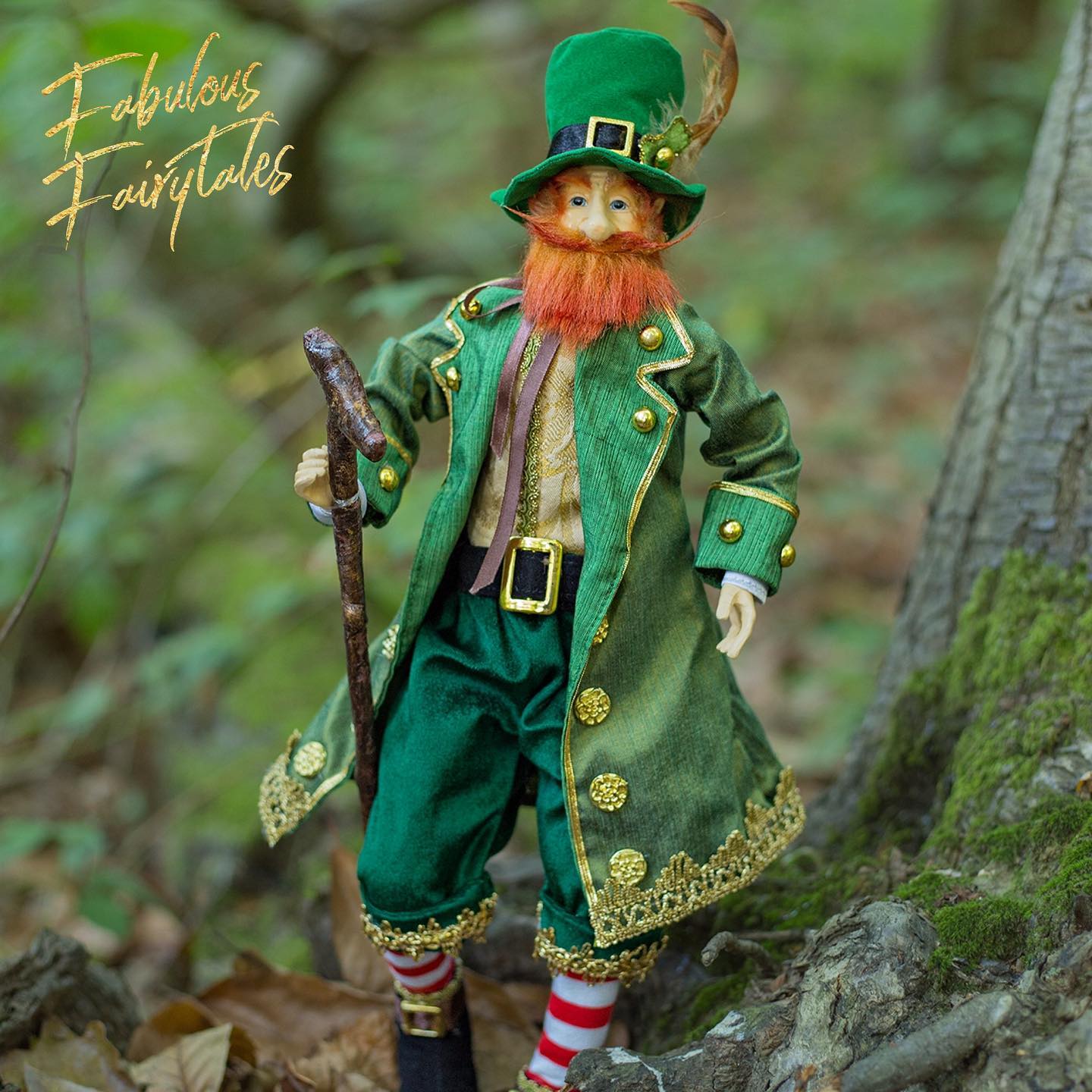The image showcases a detailed figurine of an Irish leprechaun, depicted with classic features and attire. The leprechaun sports a vibrant green ensemble including a top hat adorned with a brown feather, a jacket with golden ornaments and buttons, green trousers, and a black belt with a prominent buckle. His facial hair—a long, red beard and mustache—adds to his whimsical appearance. Completing his outfit are striped white and red stockings and black shoes. He holds a black cane, enhancing his dapper look. The scene appears to be a miniature forest setting, with the leprechaun poised as if strolling past a model tree trunk dotted with patches of green moss. Overhead, in the top left corner, the words "Fabulous Fairy Tales" are elegantly inscribed in gold, cursive writing, emphasizing the enchanting and stylish Irish folklore theme suitable for a St. Patrick's Day celebration. The figurine stands around 10 inches tall, giving it a prominent presence in the scene.